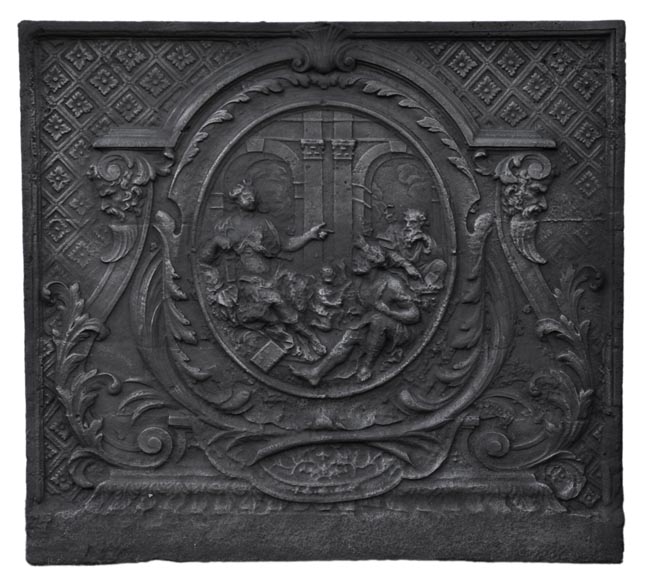The image depicts an intricately designed piece of art, likely crafted from iron or metal, with a detailed, stone-like texture. At the center, there's an oval or circular window showcasing a scene reminiscent of a knight’s or king’s court. Within this centerpiece, a man adorned with a crown stretches his arms outward, standing on the left. To the right, another man sits in the background, while a third figure, possibly a child, is positioned in the foreground. The background reveals architectural elements like archways, suggesting an ancient setting, potentially Roman in style. Surrounding the central scene is a framework decorated with elaborate scrollwork and foliage, leading to additional ornate patterns, including a flower motif etched into the stone-like material. The overall design is richly detailed, blending Baroque elements with a sense of timeless regality.